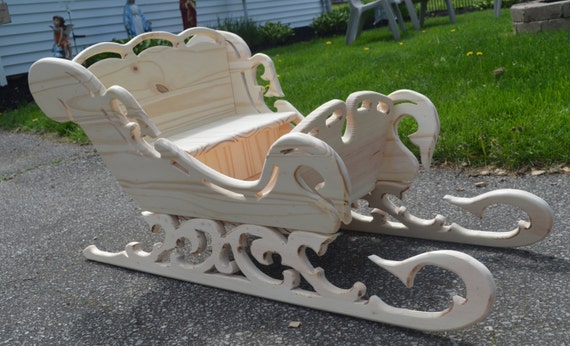The image depicts a large, unfinished wooden sleigh reminiscent of Santa Claus's sleigh, positioned outdoors on what appears to be a driveway made of blacktop or asphalt. The sleigh, crafted from light-colored, sanded wood, features ornate, embellished blades with front edges that curve into serif points. The sleigh includes a seat that seems to accommodate two people. Surrounding the sleigh, on the right side, is very green grass dotted with yellow flowers. In the background, a house with white siding is visible, along with a variety of outdoor ornaments and statues. Notably, there are statues of the Virgin Mary dressed in white and blue, a fairy girl sitting on a mushroom, and possibly an angel or Jesus. Nearby, the bottom halves of some plastic deck chairs are visible, along with what appears to be bricks forming a small structure, possibly a pond. The entire scene is bathed in outdoor daylight, capturing a peaceful and detailed yard setup.